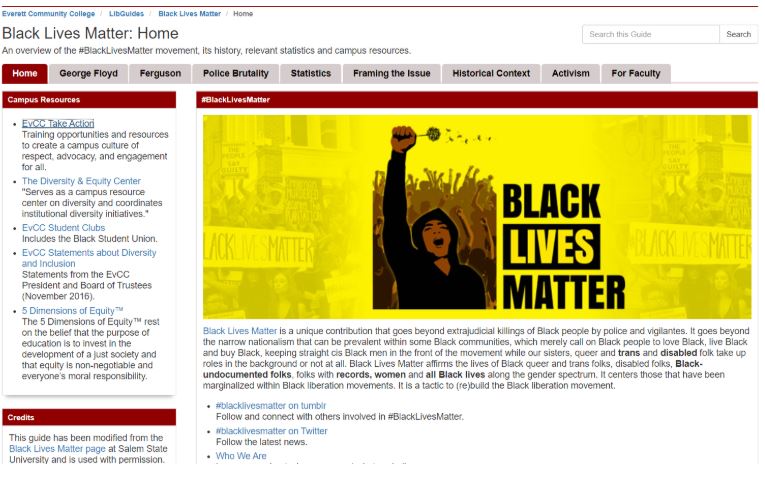Screenshot of a web page from Everett Community College’s LibGuides dedicated to the Black Lives Matter movement. The browser window displays the website, characterized by a clean and contrasting color scheme of white, red, and yellow. At the top of the page, navigational breadcrumbs outline the path: Everett Community College > LibGuides > Black Lives Matter > Home. The page is titled "Black Lives Matter: Home," followed by a subheader summarizing the page content: "An overview of the hashtag Black Lives Matter movement, its history, relevant statistics, and campus resources."

In the top right corner is a search bar labeled "Search this Guide," accompanied by a search button to facilitate finding specific information. Navigation tabs arrayed across the top of the page include Home, George Floyd, Ferguson, Police Brutality, Statistics, Framing the Issue, Historical Context, Activism, and For Faculty. The Home tab is marked in red to signify selection.

On the left sidebar, sections labeled "Campus Resources" and "Credits" provide additional links for further exploration. Dominating the right side of the page is a vivid yellow graphic featuring the words "Black Lives Matter" and an illustration of several people raising their fists in solidarity. The central figure in the image is depicted in black attire against a yellow monochrome backdrop. Below the graphic, there is informative text about the Black Lives Matter movement.